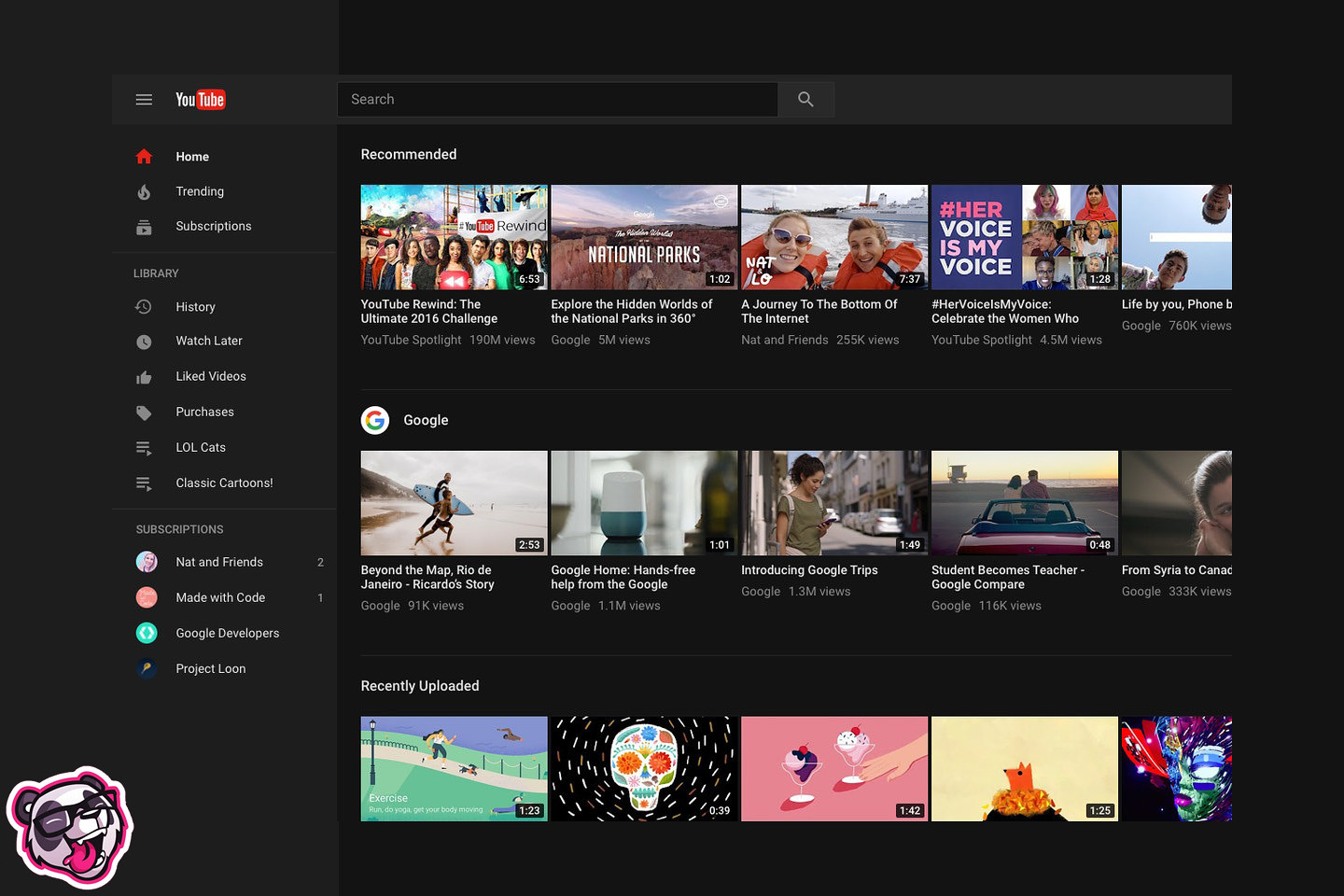The image depicts a YouTube application interface displayed in dark mode, with a black background dominating the screen. In the upper left corner, the iconic YouTube logo is visible, along with the standard sidebar options including Home, Trending, Subscriptions, History, and Watch Later. The main content area is organized into three horizontal rows of video thumbnails: the top row showcases recommended videos, the middle row features content related to Google, and the bottom row highlights recently uploaded videos.

In the lower-left corner of the screen, there is an interesting element adding a touch of personality to the setup—a sticker, or possibly a screen decoration, of a cartoon dog. This whimsical character has a gray face with a white nose and white markings around the nose. It is wearing black plastic-framed glasses and has its mouth open wide in a joyful smile, revealing a pink tongue lolling out. The sticker is outlined with a pink border, which is further accentuated by an additional white border, making the playful image stand out against the dark mode backdrop.